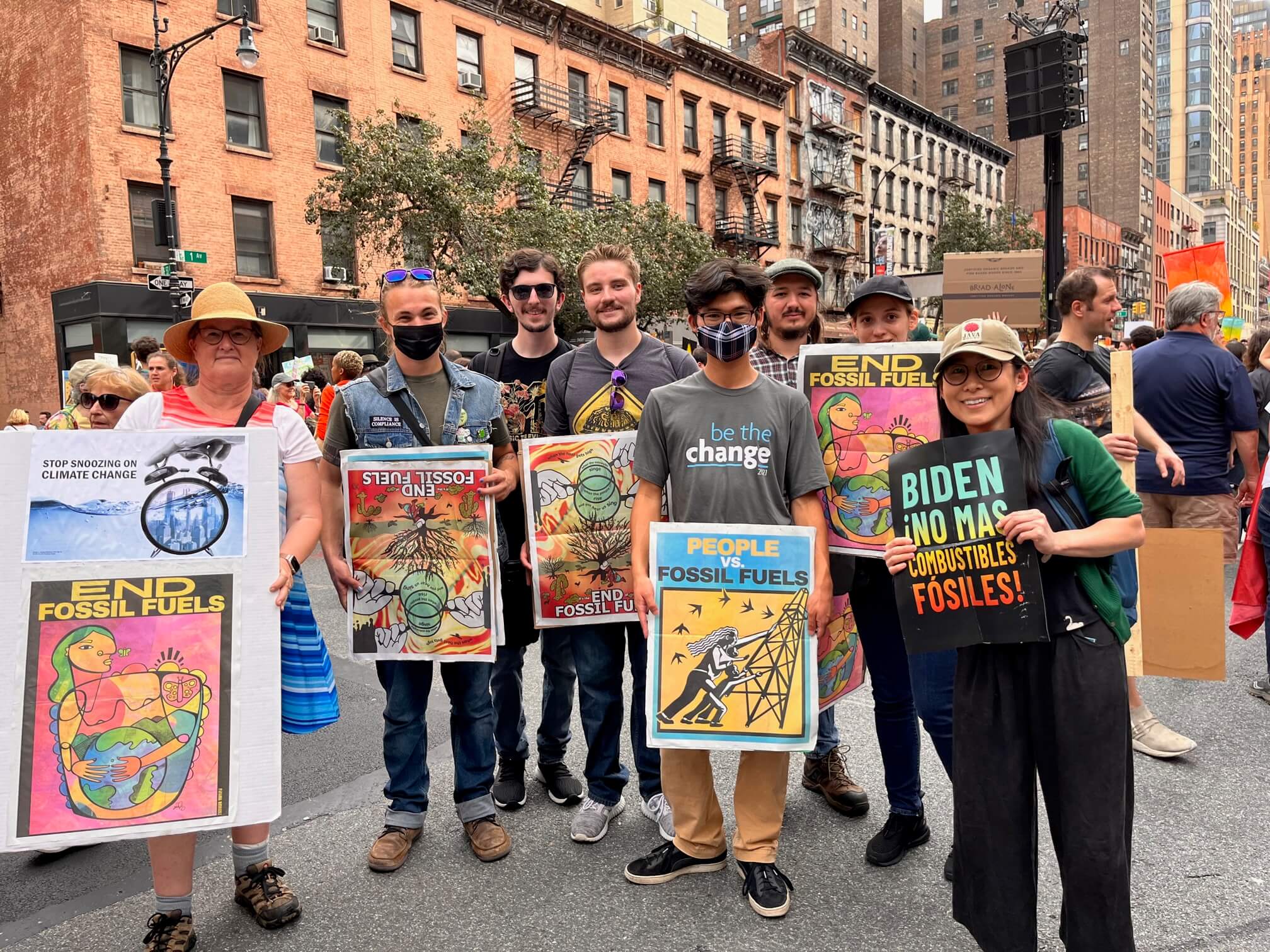In this detailed outdoor image, we see a group of around a couple dozen protestors—primarily younger individuals, with a few older ones—standing on a gray sidewalk in what appears to be a large city. The backdrop includes diverse high-rise buildings of varying colors and shapes, with reddish-brown structures to the left and taller gray and beige ones to the right, further reinforcing the urban setting. The protestors are holding up a variety of signs aimed at raising awareness about climate change and fossil fuels. Notable signs include: "Stop Snoozing on Climate Change," "End Fossil Fuels," and "People Versus Fossil Fuels." One protestor has a sign held upside down that reads "End Fossil Fuels," while another nearby holds the same sign right side up. A central figure wearing a shirt emblazoned with "Be the Change" stands in the middle, displaying a sign with "People Versus Fossil Fuels" and an image of people toppling an oil rig. On the right, a girl holds a sign that says, "Biden, No Mas Combustibles Fossils," with a woman in a green sweater, dark pants, and a blue hat prominently displaying a similar message. The scene is lively and colorful, showcasing the protestors' diverse attire and united spirit in advocating for environmental action.